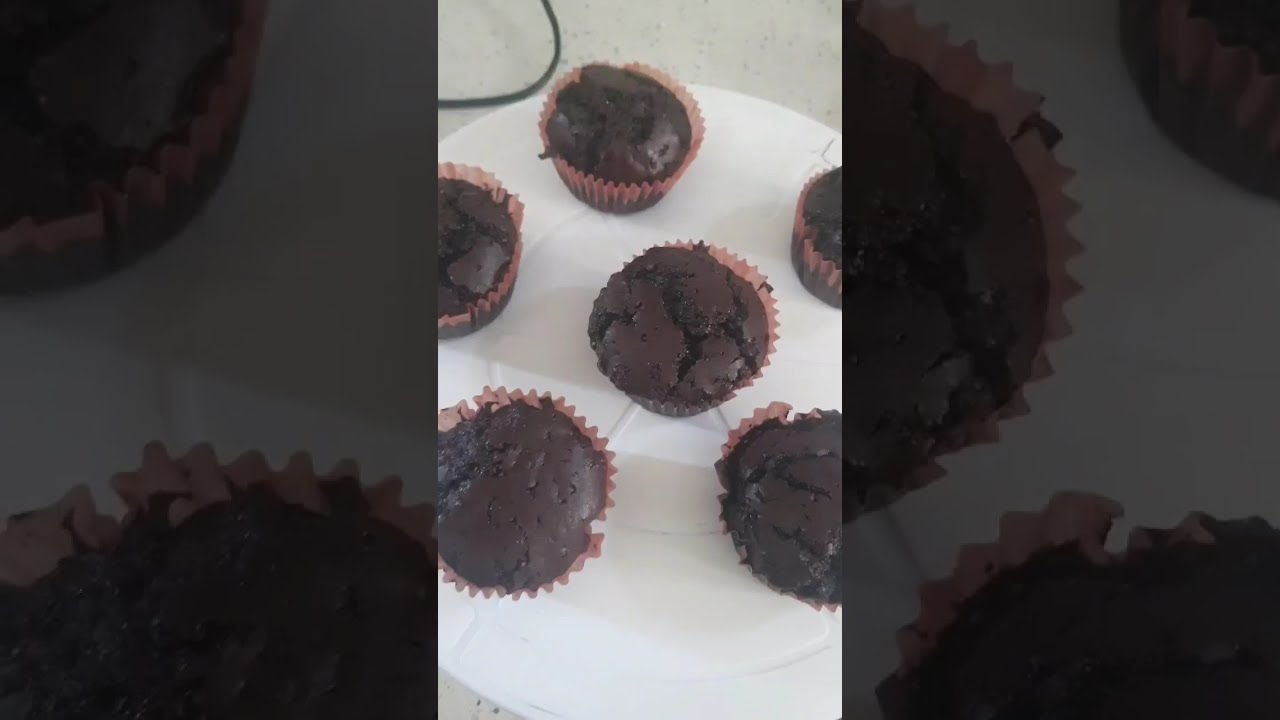This top-down image shows six freshly baked chocolate cupcakes arranged in a circular pattern — one in the center and five around it. The cupcakes are nestled in light brown or light red paper wrappers, giving the impression of rich, moist brownies. They are placed on a white, flat, round tray that seems to be a rotatable cake turntable, commonly used for cake decorating and baking purposes. The surface of the tray is segmented slightly with faint lines, and there's a visible black cord in the upper left corner, hinting at the casual, homey setting of the photo. Additionally, the left and right edges of the image are bordered by an enlarged, blurred version of the same image, creating a unique framed effect. Some cupcake tops appear cracked and slightly bulging while others are smoother, adding to the rustic charm of the freshly baked confections.